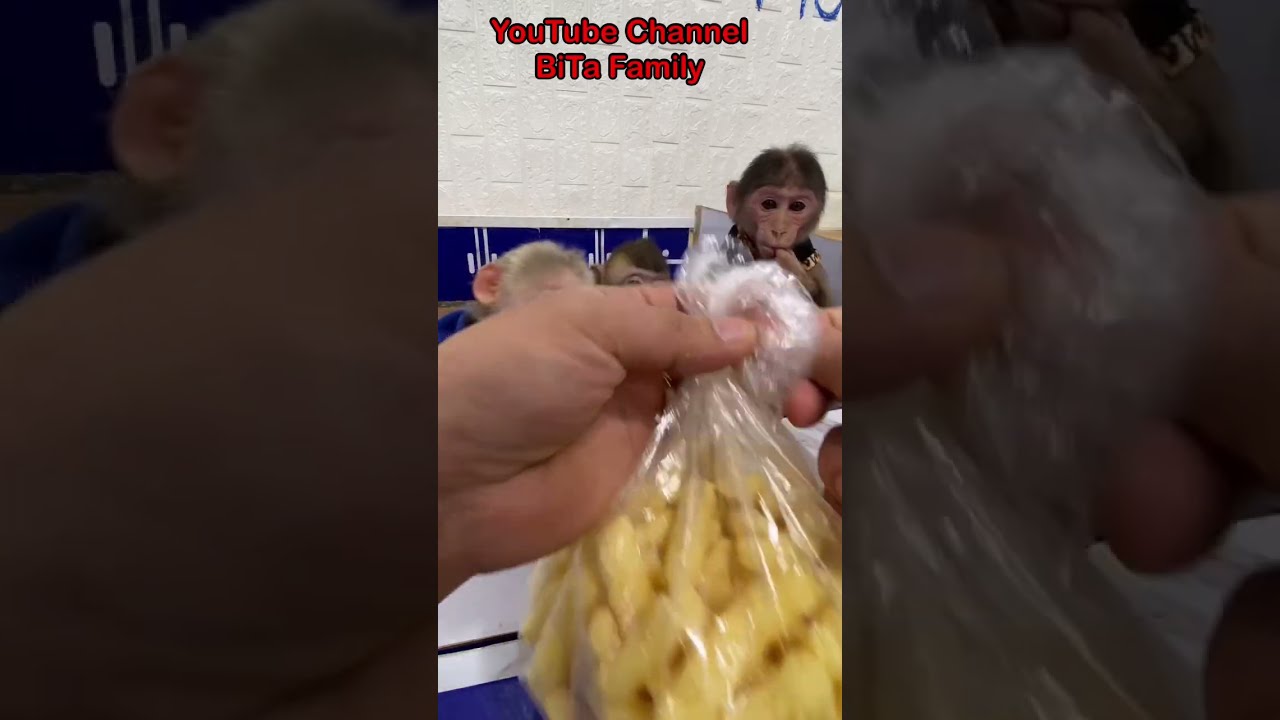This photograph, framed within faded vertical borders created by enlarged, darkened versions of itself, features an up-close view of a left hand, presumably of Caucasian descent, holding a clear plastic bag filled with golden crinkle-cut French fries. At the top center of the image, text in red reads "YouTube channel" with "Beta Family" just below it. The text is outlined in black. The background showcases a beige wall and a white painted cement block wall with a blue border at the bottom. Positioned between the hand and the wall, three monkeys sit on a counter. The prominent monkey, with brown fur, gazes directly at the camera, seemingly expectant. The other two monkeys are partially obscured by the hand holding the French fries, adding a sense of curiosity and interaction to the scene.